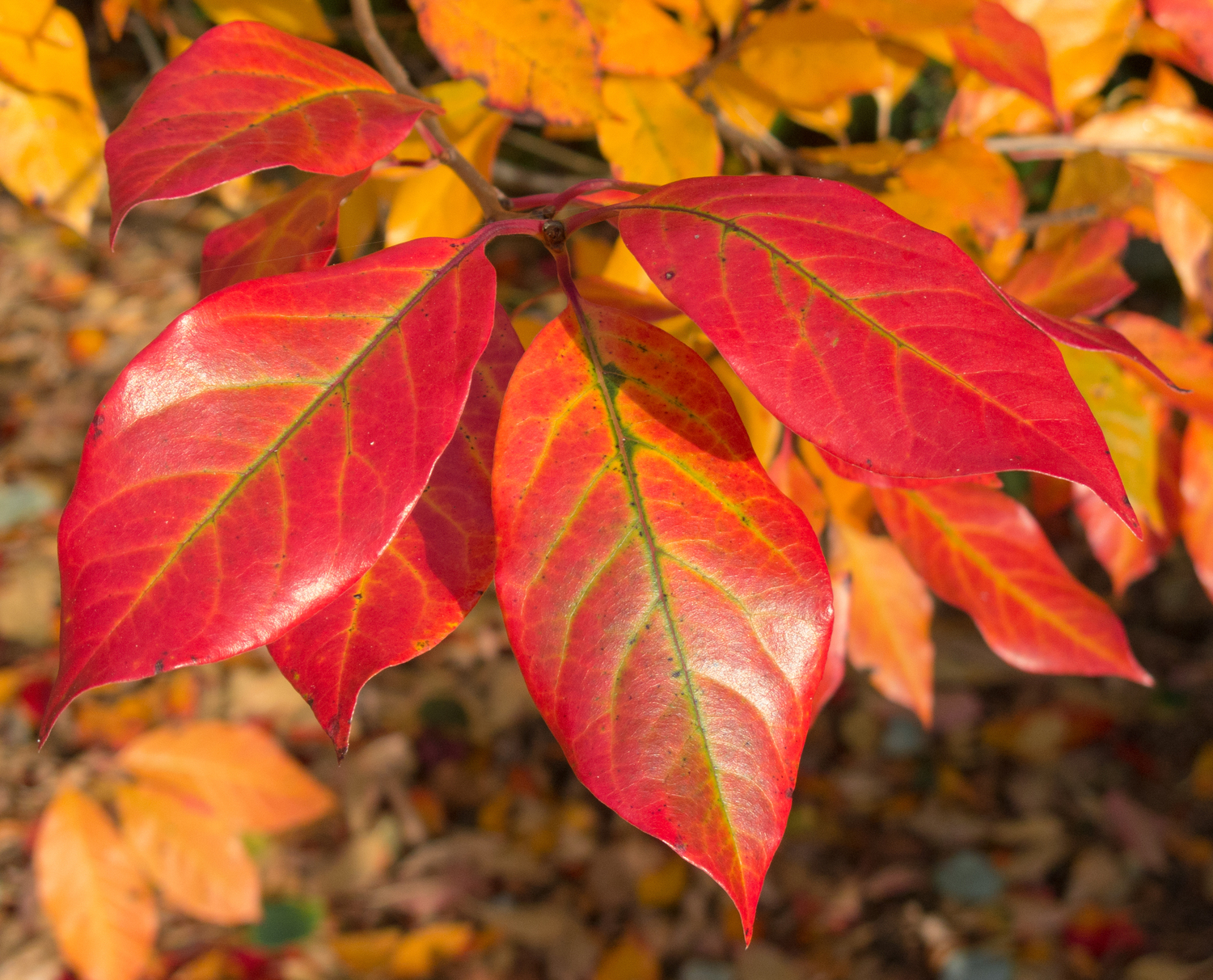This photograph captures the vibrant beauty of autumn with a close-up of a clump of multicolored oval leaves. Dominating the frame are three bright red leaves, adorned with intricate yellow veins and green centers, creating a striking contrast. Surrounding them are additional leaves in shades of orange, yellow, and brown, some of which appear to have just fallen to the ground. The detailed focus highlights the red leaves, while the blurry background of fallen leaves and distant trees suggests an outdoor setting during fall. The image is square-shaped, and you can notice a branch extending from the top, supporting the cluster of vibrant leaves. Shadows from the upper leaves cast interesting patterns on the main leaf in the center, enhancing the depth and texture of the scene.